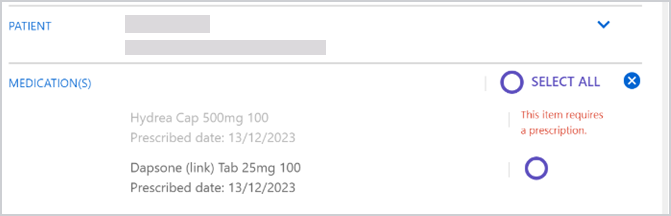The image shows a white-background document from a site displaying patient information and prescribed medications. The patient's identifiable information, spanning two lines, has been redacted with a gray box. The first line is shorter, while the second, likely the address or ID number, is significantly longer. Below this redacted section, the document lists two medications:

1. **Hydrea Cap**: 
   - Dosage: 500 milligrams
   - Quantity: 100 capsules
   - Prescribed Date: December 13, 2023
   - Note: This item requires a prescription (grayed out).

2. **Dapsone**:
   - Dosage: 25 milligrams
   - Quantity: 100 tablets
   - Prescribed Date: Unspecified
   - No mention of prescription requirement.

Overall, the document highlights important details about the prescriptions, emphasizing that Hydrea Cap necessitates a prescription, while it's unclear if the same applies to Dapsone.